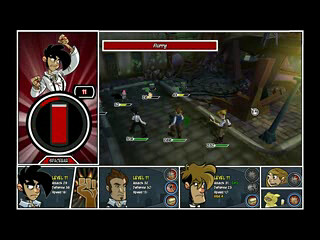This image captures a scene from a video game, featuring anime-style characters. The scene appears to depict a maze or labyrinth set in a dark, urban environment. A streetlamp partially illuminates the area, casting a dim light on the surroundings. Below the main scene, a series of five to six different characters are displayed, presumably the characters present in the game. A red banner runs across the top of the image, though the text on it is unreadable. The overall atmosphere suggests a mysterious or challenging gameplay experience within an anime-inspired world.